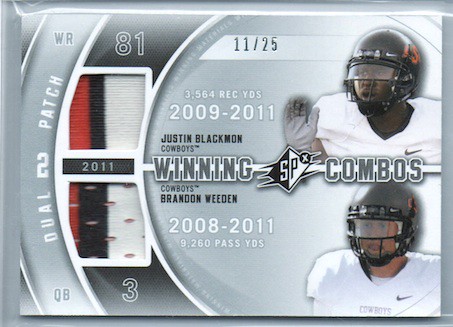The image is a sports card with a gray background featuring two football players, Justin Blackman and Brandon Weeden, both from the Oklahoma State Cowboys, not to be confused with the Dallas Cowboys. The card presents a visually split layout with Blackman on the top half and Weeden on the bottom. Blackman’s section includes his stats: 3,564 receiving yards from 2009-2011, and his jersey number 81. Weeden's section notes his passing yards: 9,260 from 2008-2011, alongside his jersey number 3. Both players are shown wearing black helmets with orange or red accents. The card prominently features "Winning Combos" and "11/25" indicating it’s part of a limited edition series. On the left side, the details "QB" for Weeden and "WR" for Blackman are displayed, along with two cutout patches, possibly pieces of their jerseys.